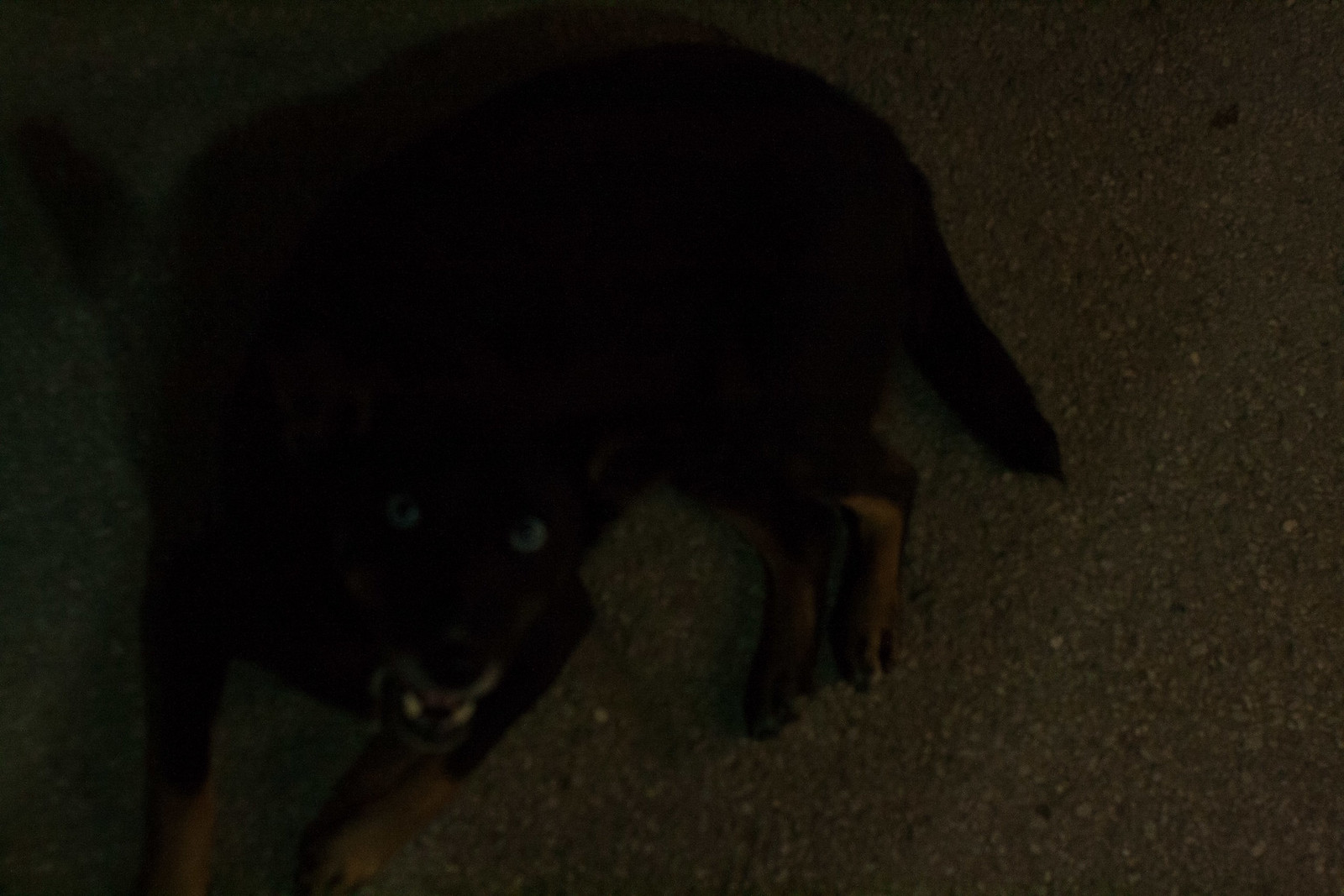In this photograph, the viewer is given a bird's-eye view of a black dog laying on a concrete surface. The dog, which features a striking combination of black and tan fur on its legs, is positioned in such a way that it appears to be looking directly up at the person taking the photo. The dog's blue eyes, which seem to pierce through the photograph, add an intense and eerie element to the image. Despite the somewhat sinister appearance given by the visible two teeth, the dog seems to be wearing a subtle smile. The dog's full body is captured in the shot with the exception of one front paw, which is just out of the frame, while the remaining three paws are clearly visible. The dim lighting accentuates the dark fur and creates a mysterious ambiance, making the image both captivating and slightly unsettling.